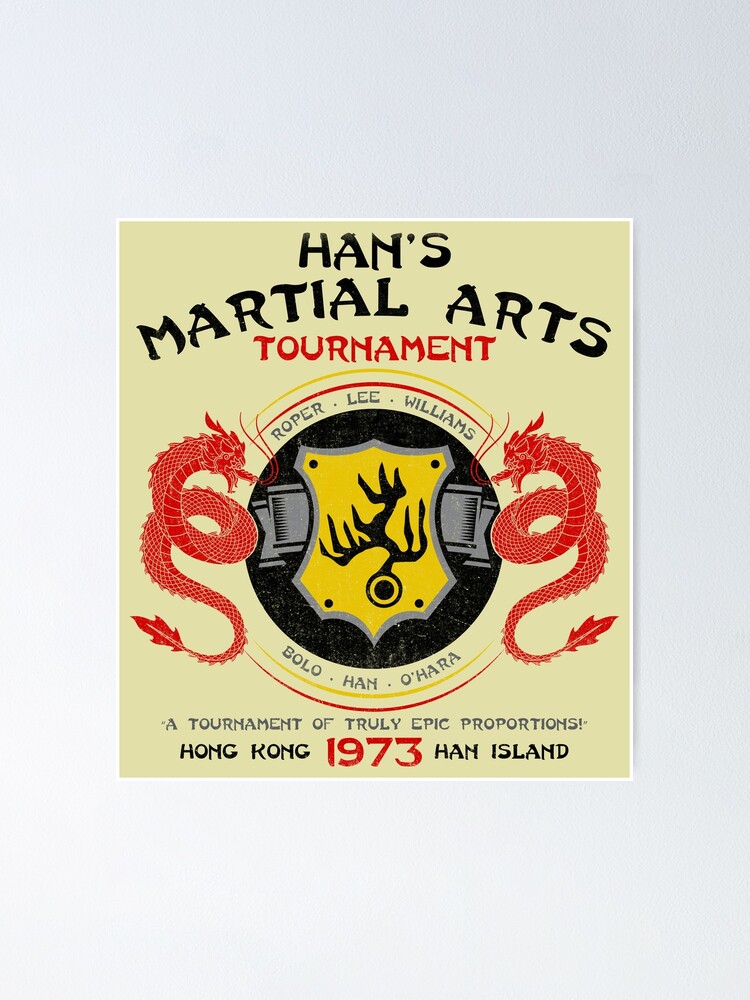This vivid poster from Han's Martial Arts Tournament, set against a light yellowish-green background, captures the essence of an epic showdown held on Han Island in Hong Kong, 1973. Bold and easy-to-read script prominently features the names: Roper, Lee, and Williams at the top in a slightly curved arc, while Bolo, Han, and O'Hara are displayed similarly at the bottom. Central to the design is a striking round emblem, resembling a gold badge with an abstract, possibly Asian-inspired design, flanked by two red dragons that face inward toward the emblem. The top headline declares "Han's Martial Arts Tournament" in black lettering, while "TOURNAMENT" stands out in red capital letters. Beneath the emblem, a tagline heralds "A Tournament of Truly Epic Proportions!" in bold text. All lettering is rendered in a combination of black, red, and gray hues, ensuring maximum visibility. The meticulous layout, sans additional watermarks or images, directs focus to its core elements, celebrating the prestigious martial arts event.